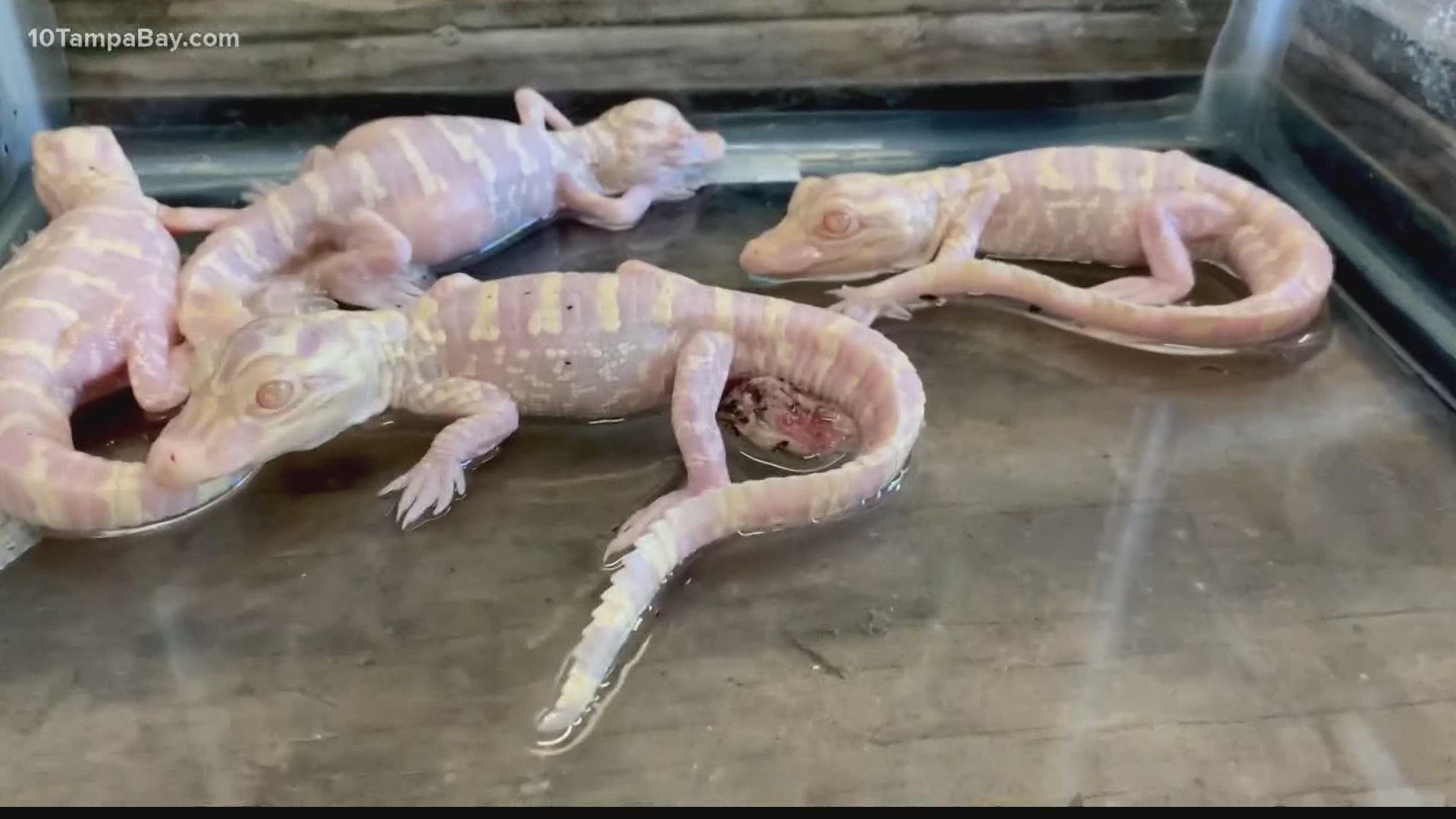This detailed image from 10TampaBay.com showcases four baby crocodiles or alligators inside a wooden, brown-colored box partially filled with water. These small reptiles appear extremely pale and translucent, possibly indicating albinism. Their delicate pink skin allows visible glimpses of their bones and blood. Accentuating their bodies are yellow lines tracing down their backs, heads, and tails. Their eyes are similarly pale, matching their flesh-toned skin. One of the crocodiles has an indistinct object attached near its tail. This enclosure and its aquatic environment suggest an acclimatization process, easing them into life outside their natural aquatic habitat.